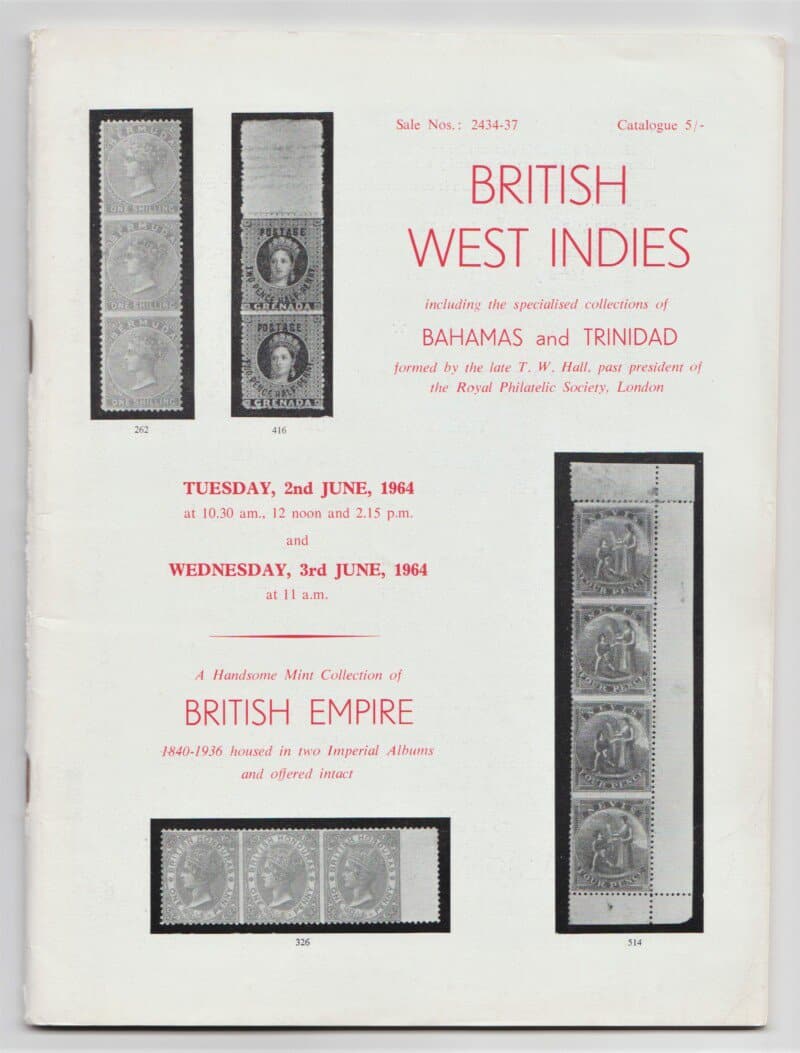This image features the front cover of an old white paper booklet secured with two staples along the spine. The cover is divided into two main sections, with a gray background. The left section showcases two columns of black and white postage stamps. The first column features three identical stamps, followed by a blank space, and two identical stamps depicting a woman with a crown. Below these stamps, there is additional text in bold:

"Tuesday, 2nd June 1964, at 10.30 AM, 12 noon, and 2.15 PM,"  
"Wednesday, 3rd June 1964, at 11 AM."

The right section of the cover contains red text, which includes:

- "Sale Number: 2434-37"
- "Catalog: 5/-"
- "British West Indies" (the largest text on the page)
- "Including the specialized collections of Bahamas and Trinidad," (in italics)
- "Formed by the late T.W. Hall, past president of the Royal Philatelic Society, London" 

Below this text, there is a bold red line. Further down, in italicized red text:

- "A handsome mint collection of British Empire, 1840 to 1936, housed in two imperial albums and offered intact."

Near the bottom, another set of stamps is displayed, consisting of three identical head bust stamps and four different stamps depicting two or three standing figures.

Overall, the booklet appears to be a catalog from a philatelic auction held on June 2nd and 3rd, 1964, featuring specialized collections of British West Indies stamps, including the Bahamas and Trinidad.